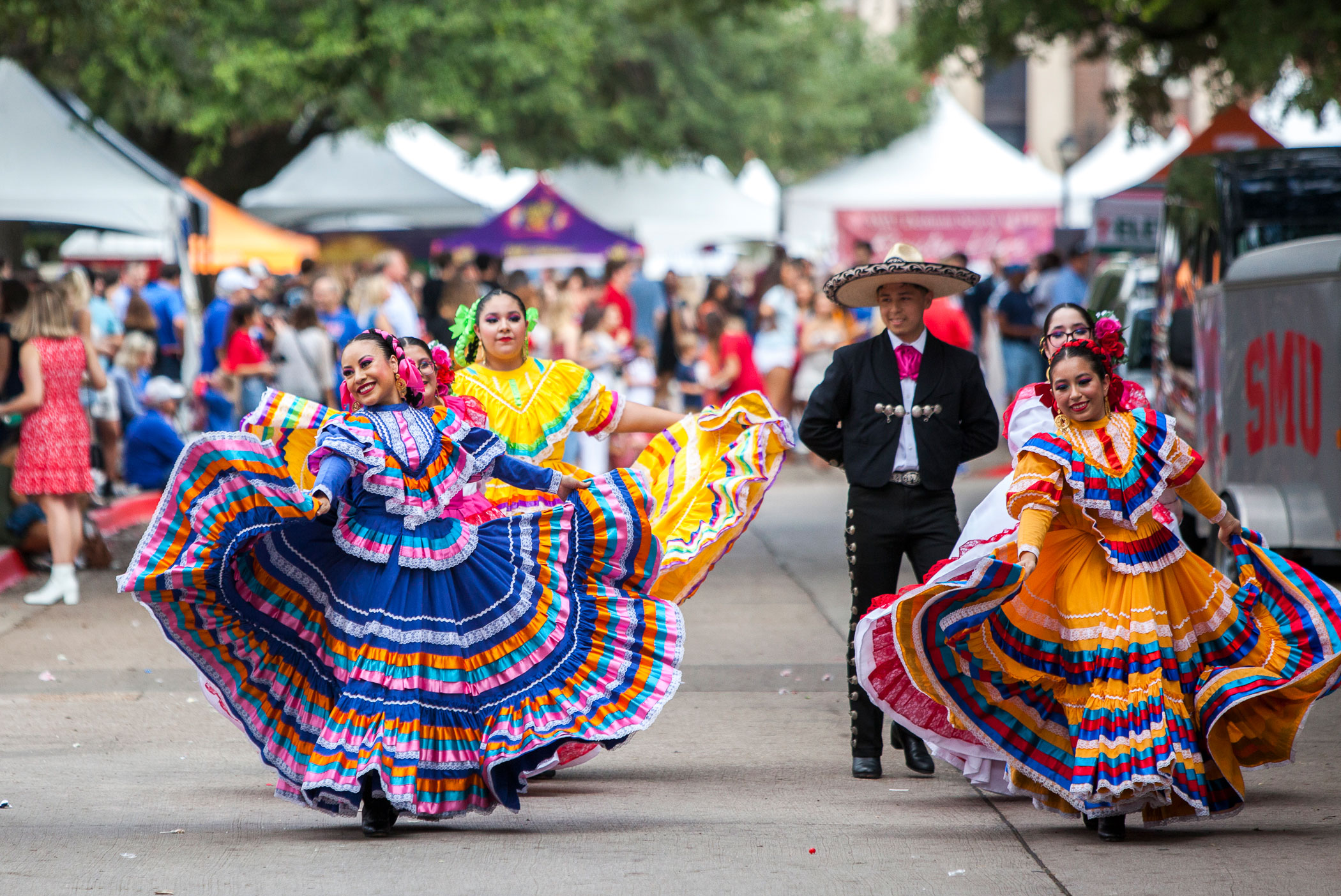This vibrant full-color outdoor photograph captures a lively street festival or parade, likely taking place in Mexico or South America, as suggested by the traditional attire and festive atmosphere. The scene centers around a man and five women dressed in traditional Mexican costumes. The man, standing slightly behind the women, wears a full black outfit with a white shirt, black pants adorned with gold buttons, a black vest, and a straw sombrero. A red tie drapes across his chest, adding to his dignified appearance. Surrounding him are five women, smiling and dancing with joy as they hold out the voluminous skirts of their colorful dresses—featuring vivid hues of blue, white, orange, teal, pink, purple, black, and red—creating a visually striking display. The women's dresses are high-necked and cover them fully, with skirts that expand dramatically when twirled.

The background of the image, although blurred, showcases bustling festival activity, with numerous tents and booths, likely food stalls and vendor booths, lining the street. Green trees and glimpses of a two-story brown building with windows frame the lively scene. There are many people visible in the background, adding to the festive atmosphere of the parade. On the right side of the photograph, a gray van with "SMU" written in big red letters can be seen, further adding to the sense of a bustling community gathering. This vivid capture encapsulates the joyous spirit and rich cultural heritage celebrated during the festival.